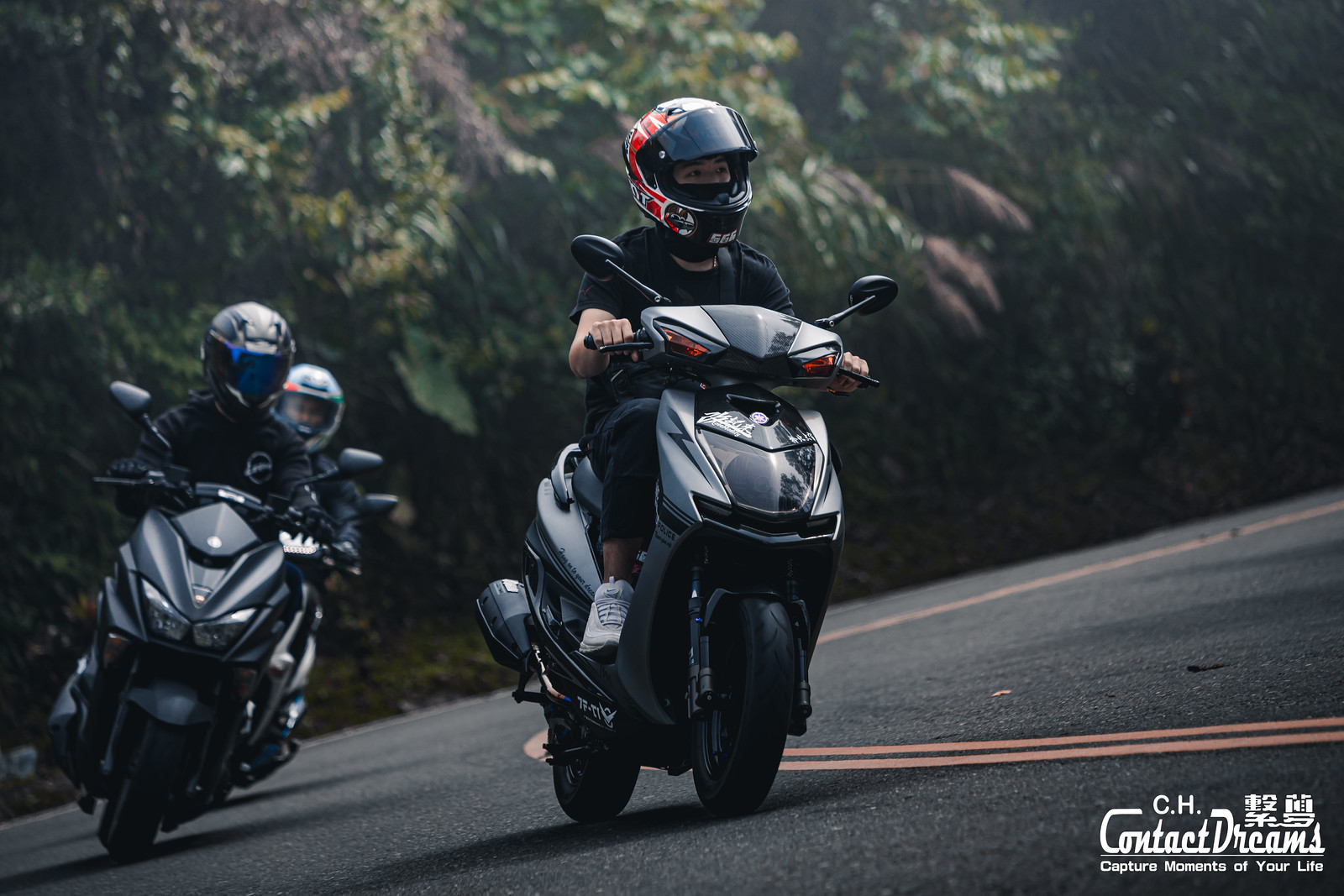In this detailed photograph, three motorcyclists are captured riding on a curvy, mountainous road surrounded by dense, dark trees. The leading rider, positioned at the front center of the image, sports a black T-shirt, a black and red helmet with an open visor revealing their eyes, and white shoes. Their motorcycle is entirely black. Close behind and slightly to the left, the second rider is fully clad in black gear, including black gloves and a black helmet, riding another black motorcycle. Further in the background, an additional motorcyclist is visible wearing a silver helmet, though the color of their bike is indistinguishable. The winding road, marked with continuous double yellow lines, indicates no passing, and enhances the scene’s sense of motion as the riders lean into the curve. In the bottom right corner, white text reads "CH contact dreams, capture moments of your life," adding a poetic touch to the dynamic image.